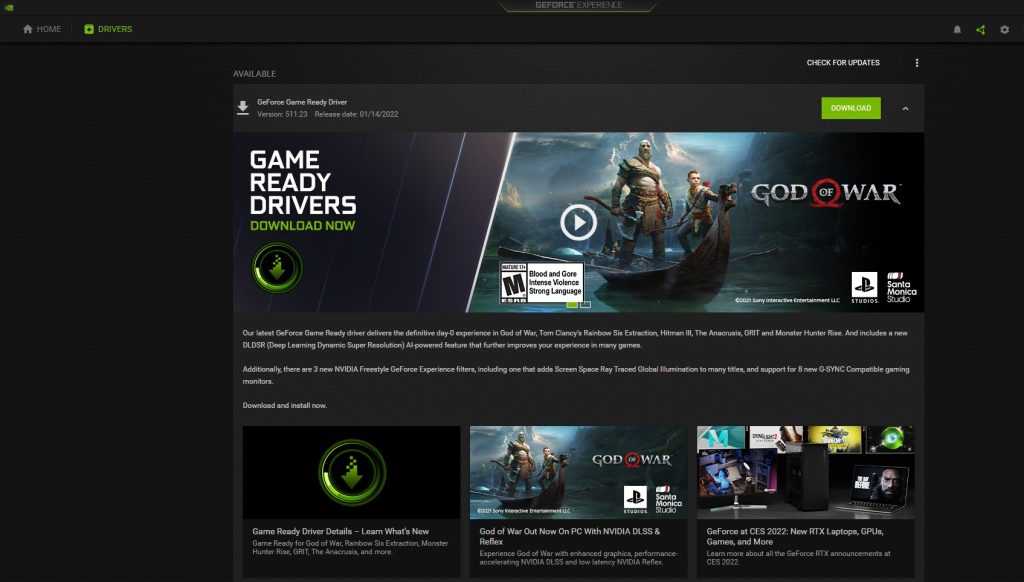The image features a user interface with a predominantly dark theme, where the left, right, and top edges are particularly shadowed. The upper left corner houses a black area beneath which the word "Home" appears accompanied by a Home icon. Below this, there is a more brightly colored green icon labeled "Drivers". Moving right, there is a green bell icon representing notifications, followed by a grey gear icon likely symbolizing settings.

In the center of the frame, there is a slightly lighter grey box. On the right side of this box, the text "Check for Updates" is displayed above an icon with three vertical dots. To the left within the box, "Available" is written in light grey letters above a downward-pointing arrow leading to a white bar containing two lines of text that are unreadable. Adjacent to this bar is a prominent green rectangle button labeled "DOWNLOAD" in uppercase white letters, featuring an up arrow.

Further to the left, "Game Ready Drivers Download" is written with an icon of a circle containing a downward arrow. This circle appears dynamic, with a fragmented tail on the arrow adding a sense of movement. To the right of this area, there are several diagonal forward slashes and a distinct box with a large "M" and a play button.

At the bottom of the interface, an image segment features two characters aboard a Viking ship with the title "God of War" indicated beneath it.